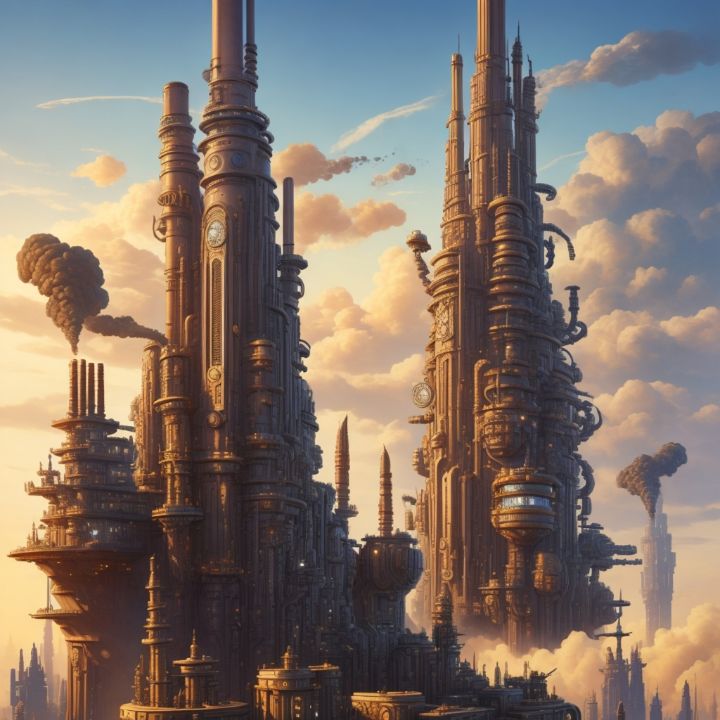This image is a digitally synthesized, steampunk-inspired city skyline featuring two prominent sets of interconnected, towering structures. The towers, predominantly copper or bronze in color, exhibit a heavily ornate and textured design, characteristic of the steampunk aesthetic. On the left side of the image, a shorter tower extends further leftward, incorporating several smokestacks that emit billowing black smoke. To the right, a collection of taller, segmented towers with various protrusions such as pipes and stacks dominate the scene.

In the foreground, the buildings are particularly detailed with rounded edges and intricate decorations. Farther in the distance, towards the bottom-right of the image, additional towers are visible, also expelling large plumes of smoke, contributing to the industrial atmosphere. The backdrop showcases a dynamic sky that transitions from a blue at the top to a golden hue towards the bottom, suggesting the approach of sunset. The sky is filled with an array of large, gold-tinged clouds, further emphasizing the towering heights of these structures, which even extend above the cloud line. Overall, the image portrays a grand, futuristic cityscape with a fantastical, steam-powered industrial vibe.